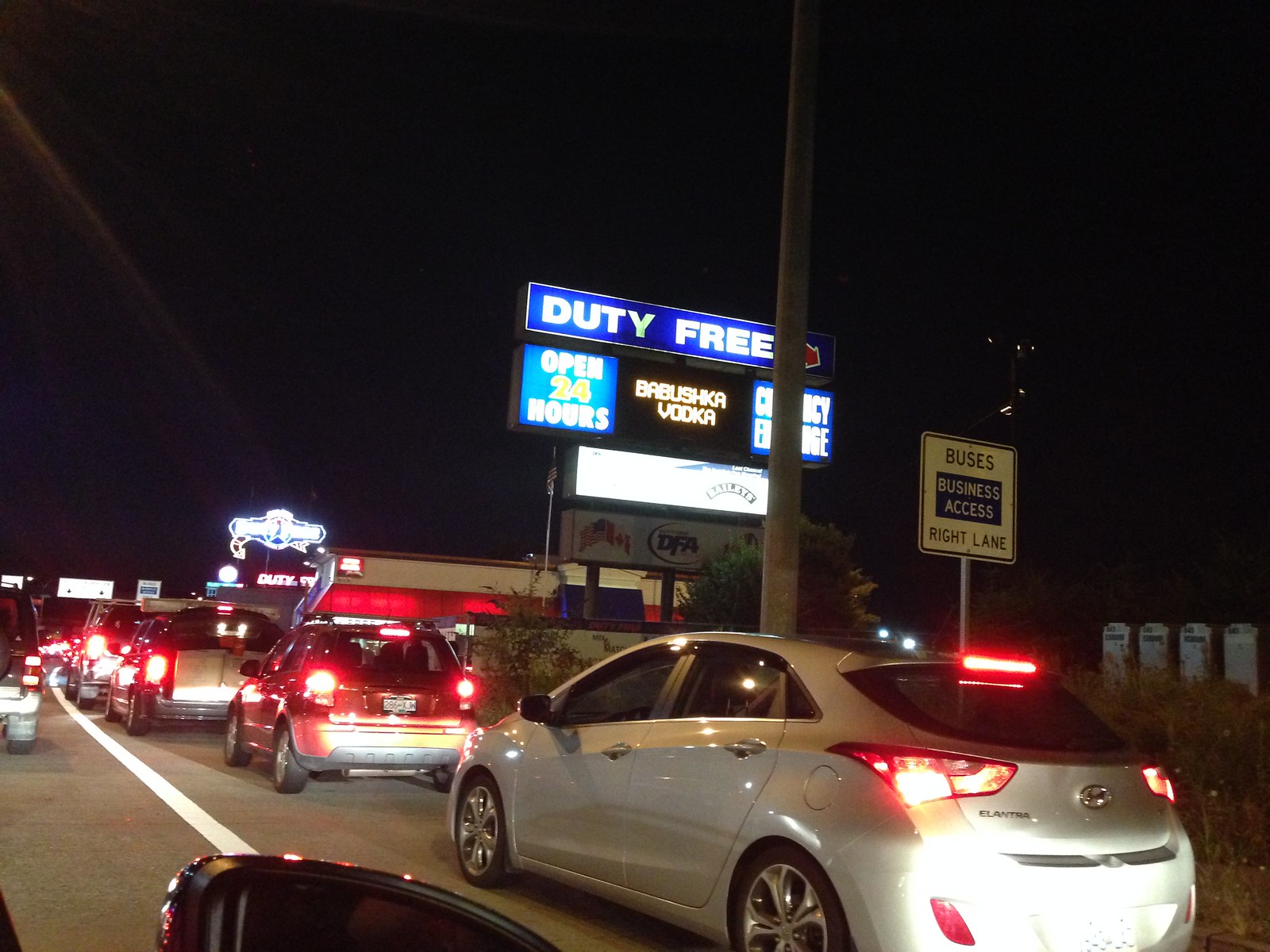This is a nighttime photo taken from the passenger side of a car, showing a scene dense with traffic. The rearview mirror is partially visible at the bottom of the frame. Ahead, vehicles are lined up, their red taillights glowing. To the left, you can see a stopped car’s taillights, while on the right, a little silver car is situated in another lane filled with traffic. Beside this silver car, there's a white road sign that reads "Buses, Business Access, Right Lane." Dominating the background is a large, illuminated business sign with multiple sections: at the top, in a blue rectangle, it says "Duty Free" with an arrow pointing downwards. Below that, in blue letters, it reads "Open 24 Hours," and in red letters, "Babushka Vodka." Part of this sign is obscured by a large concrete pole. Additionally, there are two smaller rectangular signs attached to the same pole. In the far distance, other buildings and neon signs can be seen along the street, and a black, starless sky forms the backdrop. To the right, a white building with a red awning is partly visible, along with what seems to be some port-a-potties and power lines.